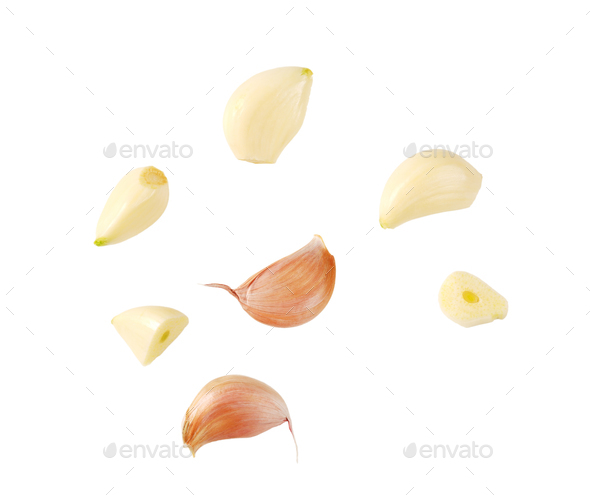The stock photograph showcases seven pieces of garlic cloves at various stages, set against a pure white background that creates a floating effect. Overlaying the entire image is a dotted gray line pattern forming diamond shapes, with sporadic semi-transparent watermarks reading "Envato." Central to the composition are two garlic cloves still encased in their pinkish outer skin, while the remaining cloves are peeled, revealing their white interiors. Positioned on the left side is a halved clove, juxtaposed by a thin slice on the right side. The cloves, including the three whole peeled ones at the top, are arranged in a seemingly random manner, offering a detailed exploration of garlic in different forms.